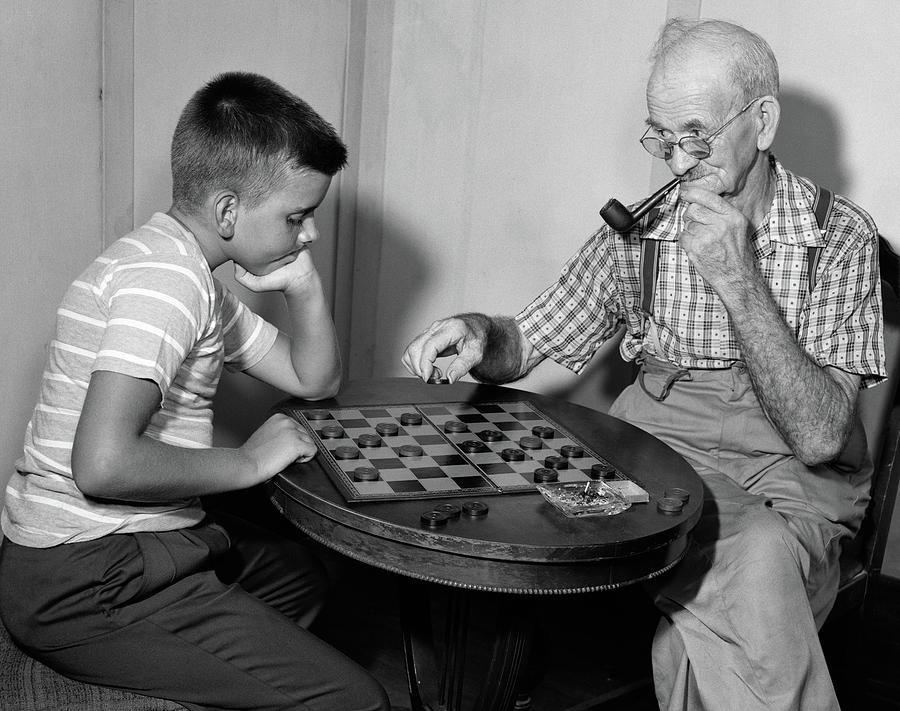This black-and-white photograph, likely taken in the 1940s or 1950s, depicts a poignant moment between a young boy and an elderly man, presumably his grandfather, engrossed in a game of checkers. The old man, with sparse hair and tinted round-rimmed glasses, sits on a chair with his legs crossed and a smoking pipe in his mouth. He wears light-colored pants, a checkered shirt with an open V collar, and suspenders. The boy, who has dark hair and a buzz cut, is seated on a stool, donning dark slacks and a short-sleeved striped polo shirt. The round table between them holds a checkerboard, checker pieces, and an ashtray. The boy intently watches the man, deep in thought over his next move, while the man gazes over his glasses at him with a mischievous expression. The background features a light and medium gray wall, adding to the timeless feel of this mid-20th-century scene.